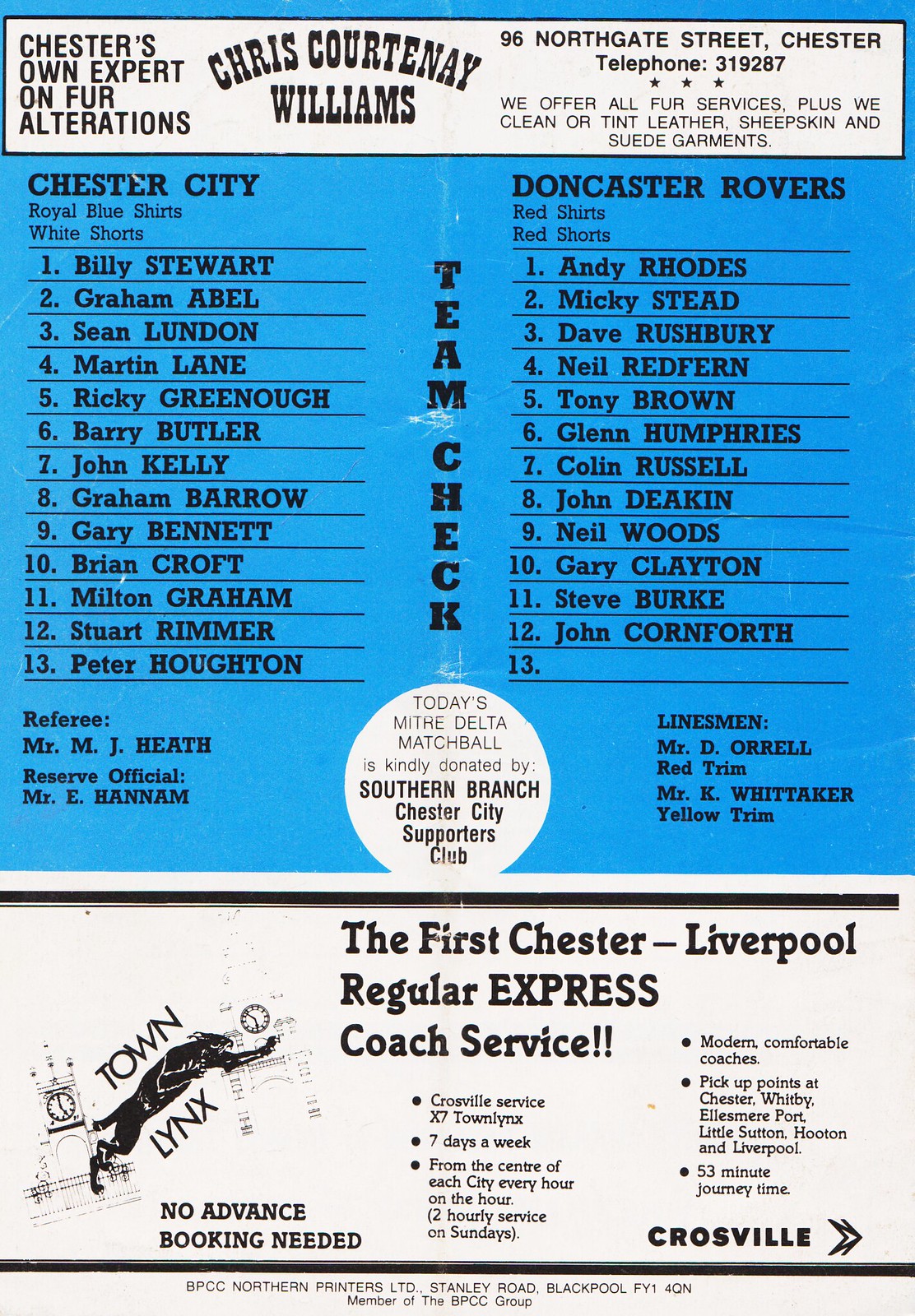The visual depicts a photocopy of a soccer pamphlet or program, expertly detailed with a structured layout. Dominating the top 60% of the image is a blue background. At the very top, a white rectangular box with a black border features an advertisement reading "Chester’s Own Expert on Fur Alterations, Chris Courtney-Williams," followed by an address, "96 Northgate Street, Chester," and a contact number, "Telephone 319287." The advertisement concludes with a star-studded note offering fur services and cleaning/tinting of leather, sheepskin, and suede.

Below this advertisement, the blue background hosts team rosters for Chester City on the left and Doncaster Rovers on the right. Chester City's section, headed by "Royal Blue Shirts, White Shorts," lists player names under "Team Check" written vertically in black. The Doncaster Rovers section, marked by "Red Shirts, Red Shorts," similarly lists players, with a tilde indicating an unlisted thirteenth name.

Between these rosters, a white circle reads "Today's Mitre Delta Match Ball is kindly donated by Southern Branch Chester City Supporters Club." To the bottom left and right of the team lists are the referee, reserve official, and linemen details.

The lower portion of the image features another advertisement in a white background, lined by black borders. It promotes "The First Chester Liverpool Regular Express Coach Service" with additional text and a picture of an animal between "Town Links." It further states "No Advance Booking Needed," with the term "Crossville" and an arrow pointing right included. Tiny print occupies the bottom margin of the poster, rounding out the comprehensive details of this soccer program.